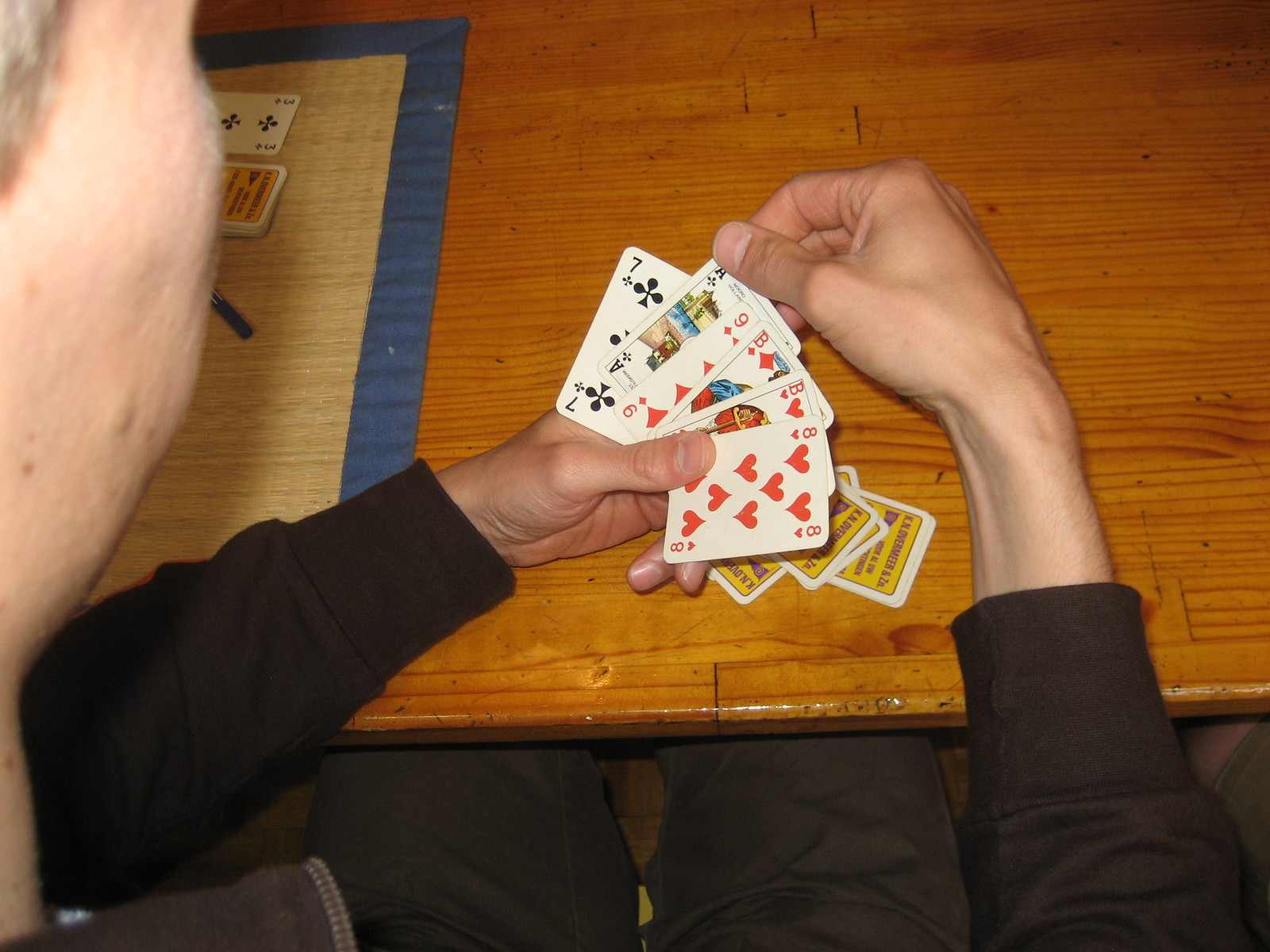A first-person perspective image captures an individual with black sleeves working with a set of playing cards on a wooden table. The person's sleeve and the side of their face are visible on the left side of the frame. In their hand, they hold five playing cards: a Seven of Clubs, an Eight of Clubs, a Nine of Diamonds, a "B" of Diamonds, and an Eight of Hearts. There are three or four cards faced down on the table that have yellow backs. The person is also wearing black pants, which are visible under the table. 

To the left side of the image, part of a play mat with a blue border and gray design can be seen. There are three clubs visible in the background near the person's face. To the right, a knee of another individual at the table is partially visible. The entire scene is indoors and shot top-down.